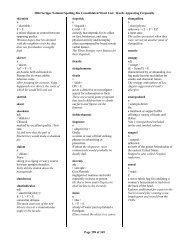The image depicts a long piece of white paper with a computer-printed layout divided into three columns of text. Each column is separated by black vertical lines. The text is extremely small and illegible, but it appears structured with bolded headings at the top of each section followed by lists or explanatory text below. From a distance, you can discern distinct segments with titles or highlighted information, indicating various topics or sections within each column. There is also a long title at the top of the page, which spans the width of the columns, and additional text at the bottom, though everything remains unreadably tiny.